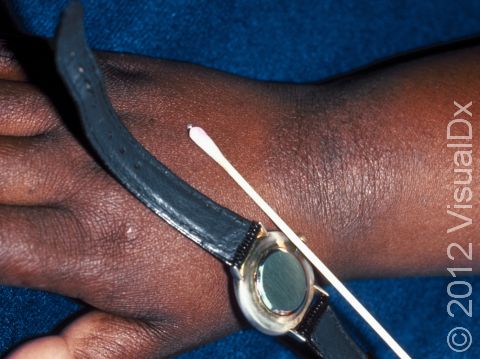In this detailed landscape photograph, a partially cropped view reveals the wrist and a portion of an African American man's hand, with fingers extending toward the left edge of the image. The hand rests palm down on a dark blue fabric background. A noticeable bruise stretches across the wrist, adding texture to the already detailed skin, which shows visible wrinkles and creases. Diagonally positioned across the back of the hand is a wristwatch, flipped inside out to expose its metal back and black leather band that curls at the ends. Alongside the watch, a long narrow white Q-tip leans against the hand, creating an intriguing composition. The watching bears the inscription "2012 Visual DX, copyrighted."